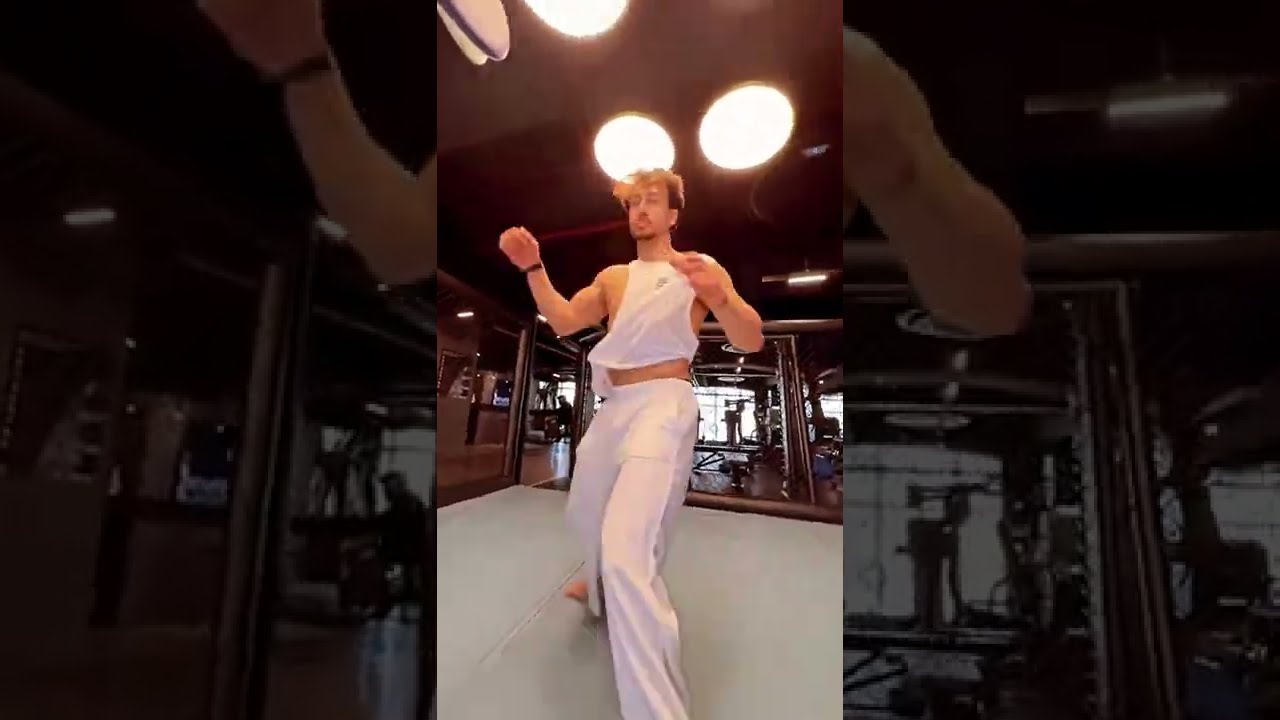The image depicts a man with light skin, orange and black hair, and a goatee, dressed in a white fitness tank top and baggy white pants, standing barefoot in a fighting ring. He strikes a pose with a wide, staggered stance, his hands up, suggesting he is either about to perform a kick or in the midst of martial arts training. The scene is brightly lit with large white lights overhead, focusing primarily on the man while rendering the background slightly blurry. Surrounding him is a blue, possibly padded mat within a cage-like structure, indicative of an MMA or karate ring. The backdrop includes a few identifiable elements such as poles, weights, and a figure on the left side, set within a gym environment. The overall image has a pixelated, video-like quality, enhancing the dynamic, action-oriented feel of the scene.